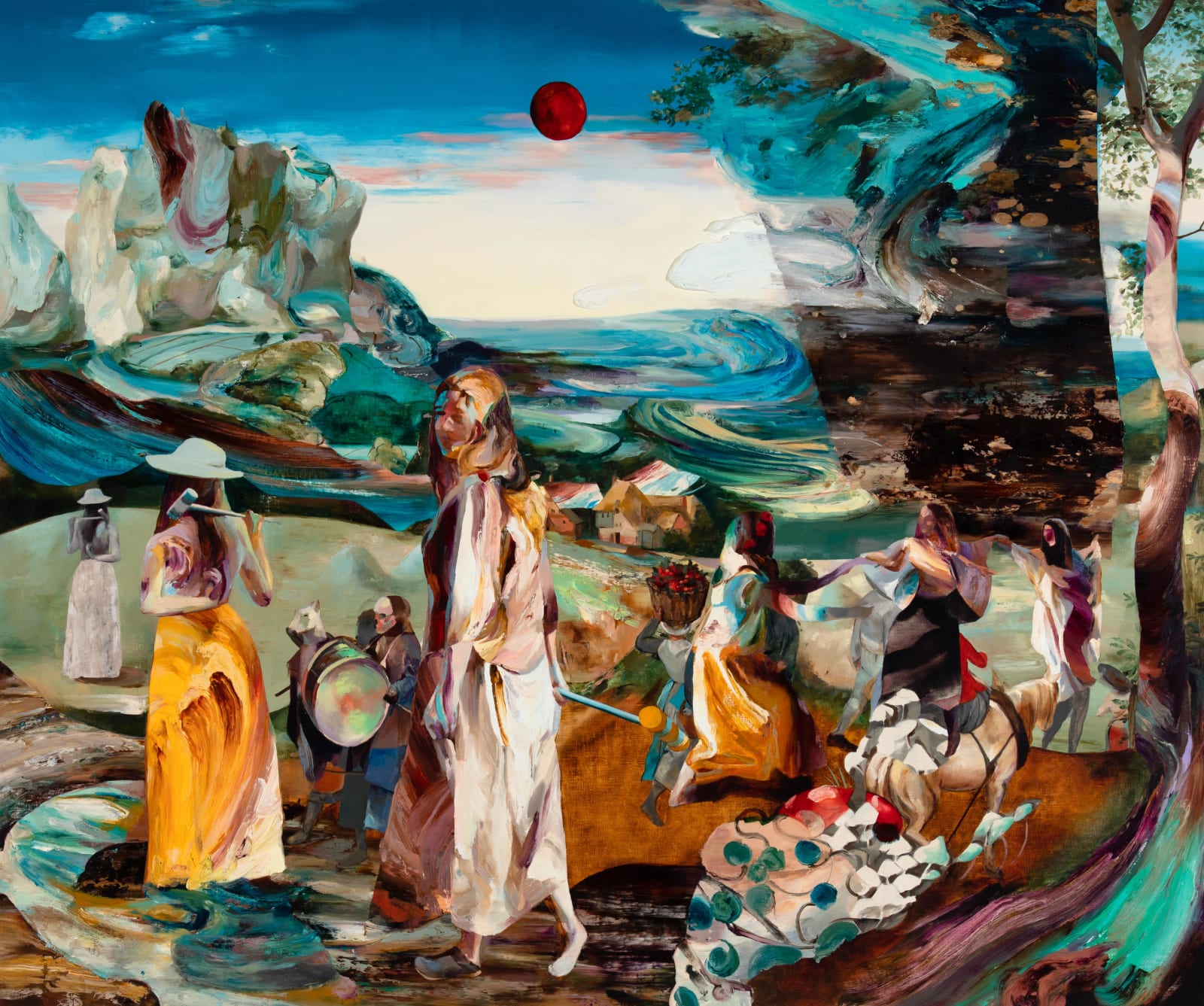In this vividly abstract painting, we are presented with a dynamic scene filled with swirling colors and various figures. Dominating the composition is a sky alive with movement, painted in vibrant blues and whites, punctuated by red spotting and a striking dark red moon or sun positioned centrally. Below this celestial display, to the left, is a cliff-like formation rendered in runny, swirled hues of light gray and brown. 

The ground beneath the figures is a dance of browns, purples, whites, and blues, creating a sense of motion and energy. In the bottom right-hand corner, a group of women, dressed in long, flowy dresses, is engaged in an array of activities. One woman, distinguished by her wicker bucket of apples, appears to blend effortlessly into the colorful whirl. Another figure, carrying a drum, shares the space with others equipped with what seem to be croquet mallets, and a few donning sun hats or Easter bonnets. 

Despite the abstract style, the figures' long hair, robes, and bare feet or sandals hint at a historical or timeless quality. A small tan horse or pack mule also makes an appearance, seemingly carrying provisions, and off in the distance, a faintly depicted building, possibly a house, sits along what might be interpreted as a shore. The scene is further complicated by the suggestion of trees or shrubbery dotting the landscape, adding layers of depth and texture to this complex, vibrant tableau.